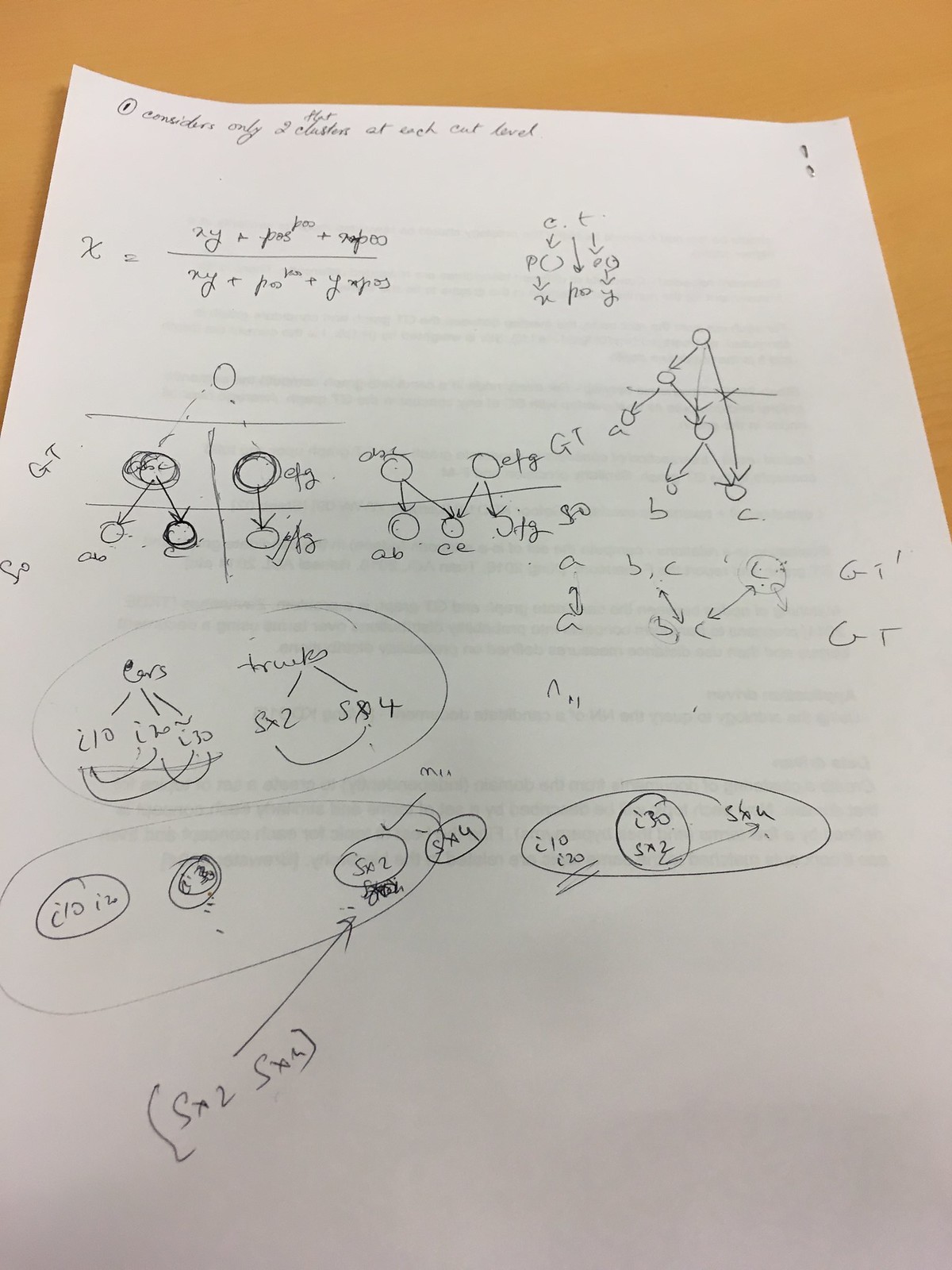The image features a white piece of paper, stapled in the top right corner. The paper is resting on a surface with a light golden-brown hue, likely a desk or table. The paper is slightly elevated on the left side, creating a subtle curve in the air.

At the top left of the paper, there are some handwritten notes beginning with the words "considers only two classes of each." Below this note, a series of equations or possibly a flowchart is situated towards the top right section of the paper.

In the center of the paper, there's a collection of symbols and letters, depicting what appear to be atoms or atomic structures. Various annotations with different symbols and letters are scattered around these illustrations.

Towards the bottom left of the paper, a segment appears to discuss "cars and trucks," accompanied by related equations and numbers. 

In the bottom center of the image, there is a final section with circled letters and numbers, featuring an equation that points to a solution marked with a checkmark.